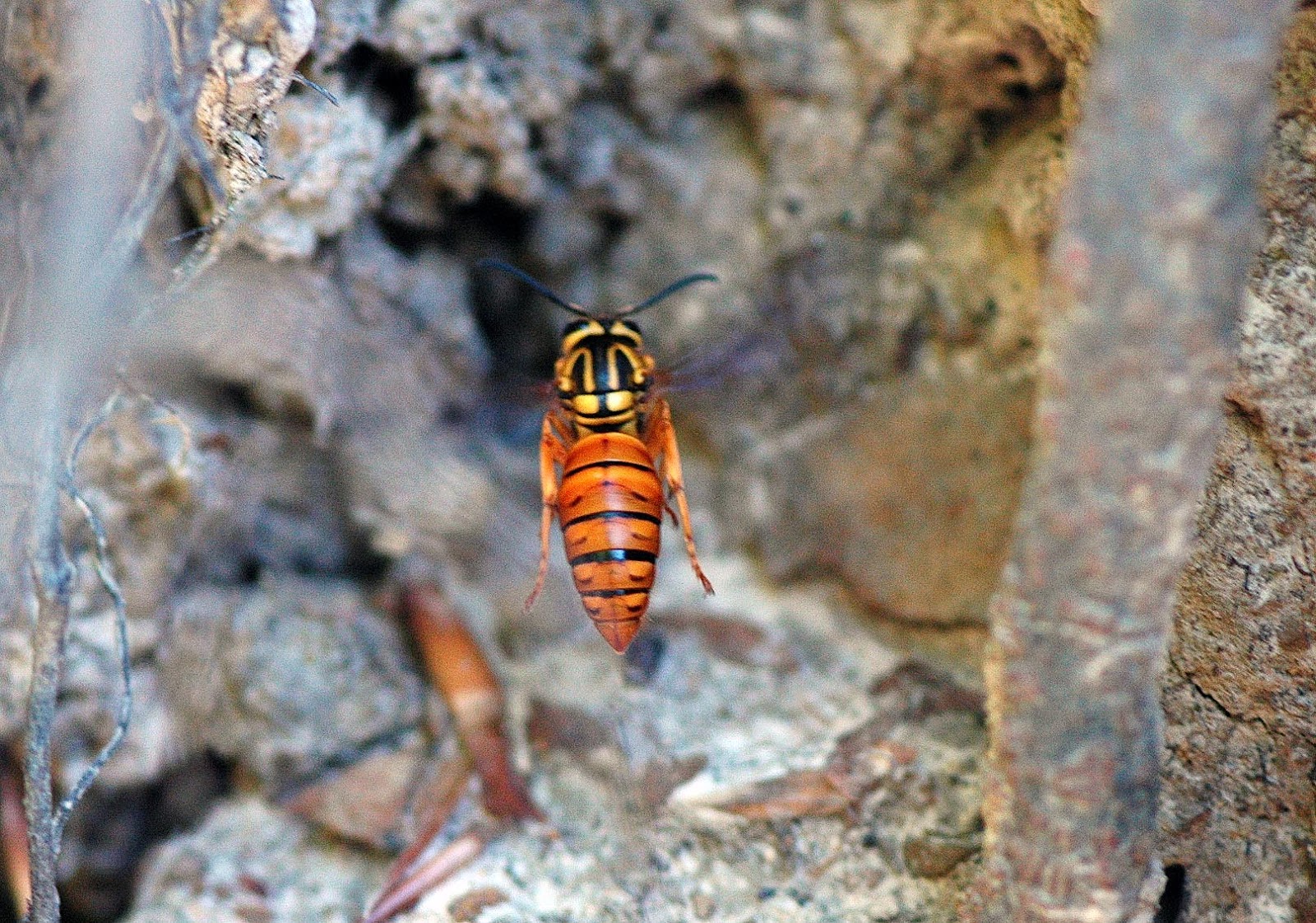The photograph captures a wasp in mid-flight, its motion blurred wings indicating either flight or a leap away from the camera. The wasp's body is bullet-shaped, with prominent features including a vibrant orange and gold lower body adorned with thin black stripes, and an upper body that transitions to yellow and black. Its head is round with two black antennae that project outwards like bicycle handlebars. The insect's cricket-like legs are thin and orange, aligning closely along its sides. The background consists of a rocky terrain, predominantly in shades of gray, pink, and brown, with visible cracks and textures suggesting stone or concrete surfaces. The composition of the photograph is horizontal, providing a detailed overhead view of the wasp against the rough, varied backdrop.